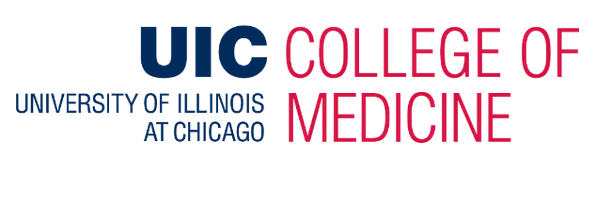A meticulously designed university logo appears in the image, seemingly sourced from the institution's official branding or website. The composition of the logo is set against a pristine white rectangular background, providing a clean canvas that enhances readability and visual appeal. The logo employs a dual-color scheme, with navy and red as its primary hues.

On the left segment of the logo, the abbreviation "UIC" is prominently displayed in bold navy lettering, immediately catching the eye. Beneath this, the text "University of Illinois at Chicago" is presented in a thinner and taller typeface, albeit at a smaller font size, maintaining the navy color for consistency.

The right segment of the logo features the designation "College of Medicine" in a striking red font. This portion of the text uses the same typeface as "University of Illinois at Chicago" but is notably larger, occupying a significant portion of the logo and emphasizing the specific college it represents. The fonts throughout the logo are sans-serif, with letters spaced closely together, contributing to a modern and cohesive aesthetic.